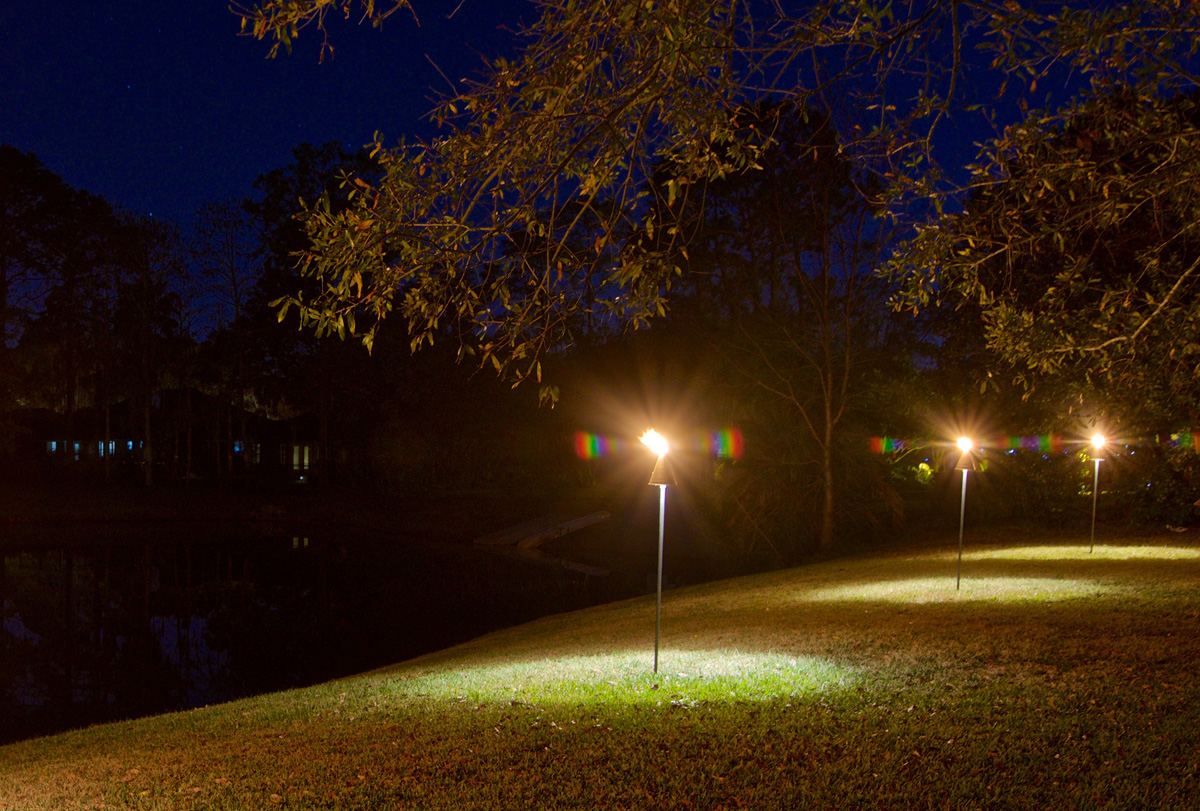The photograph captures an outdoor night scene featuring a well-maintained front yard lawn. Three garden lights, mounted on silver-gray poles, are aligned in a row positioned to the right side of the image starting from the center. These lights cast a soft, rainbow-like diffusion of beams on either side, illuminating the green grass below and creating small patches of light across the lawn. Overarching the lights are trees with lush green leaves, their branches extending into the night sky, which is painted a deep blue. In the background, there are additional trees which appear almost black against the dark sky, and some illuminated structures on the left side of the image. The yard also includes a sloping area that leads down to a dark blue body of water, resembling a lake. The overall setting emphasizes a tranquil and tastefully lit outdoor space.